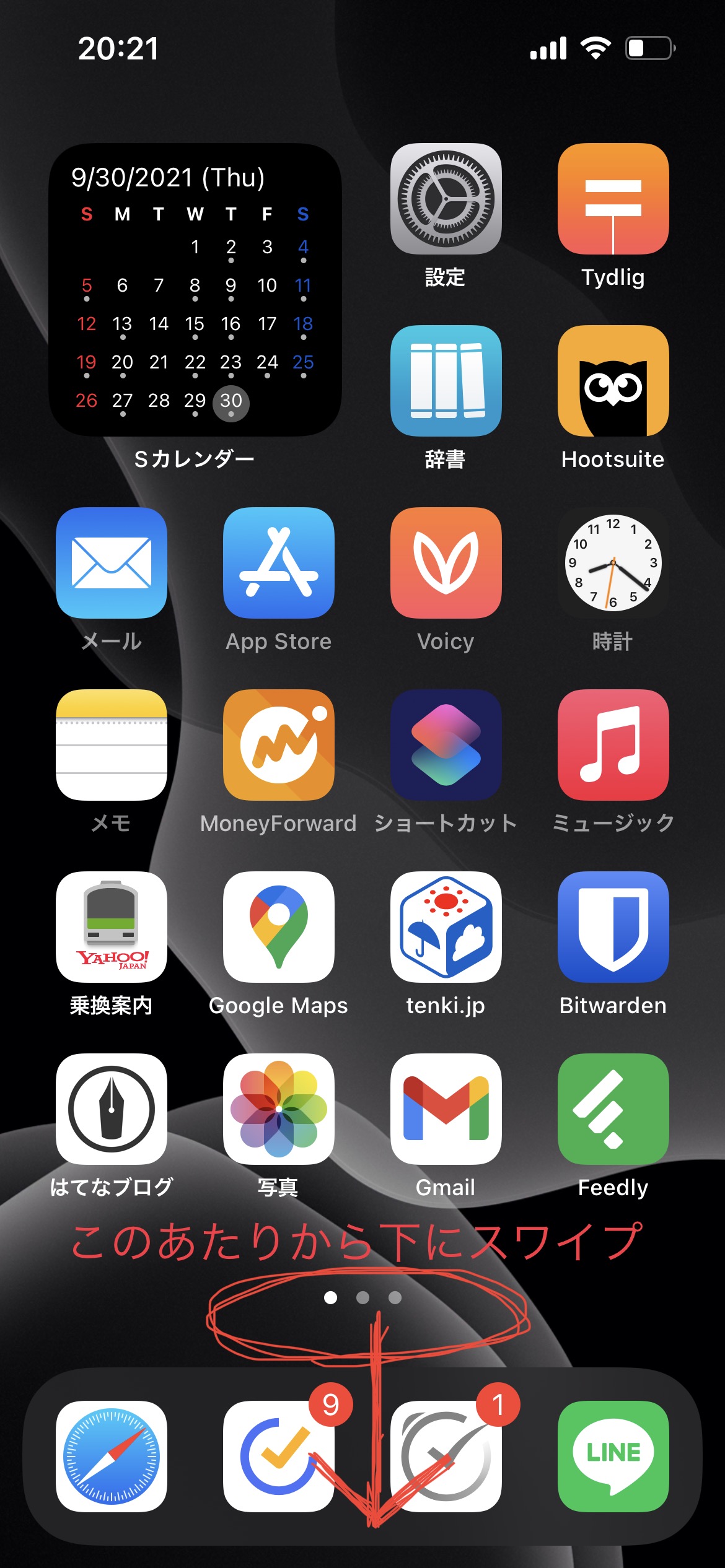The image is a screenshot of an iPhone home screen, featuring a wallpaper that is a blend of black, gray, and smoky white colors. At the top, the screen displays the time "20:21" in white text. All five bars of cell signal are fully illuminated, the Wi-Fi signal shows full strength, and the battery icon indicates approximately 25% battery remaining, marked by a white segment.

The home screen contains a variety of app icons and widgets. At the top, there is a calendar widget. The app icons include:

1. Settings
2. An app with an equal sign
3. An app featuring books
4. HootSuite
5. Mail
6. App Store
7. Voicy
8. Clock
9. Notepad
10. MoneyForward
11. Music
12. Yahoo
13. Google Maps
14. A weather app for Japan
15. Bitwarden
16. Photos
17. Gmail
18. Feedly
19. Safari browser at the bottom

At the bottom of the screen, there are dots indicating the home screen page you are on, with Japanese text or characters circled in red and an accompanying red arrow pointing downwards.